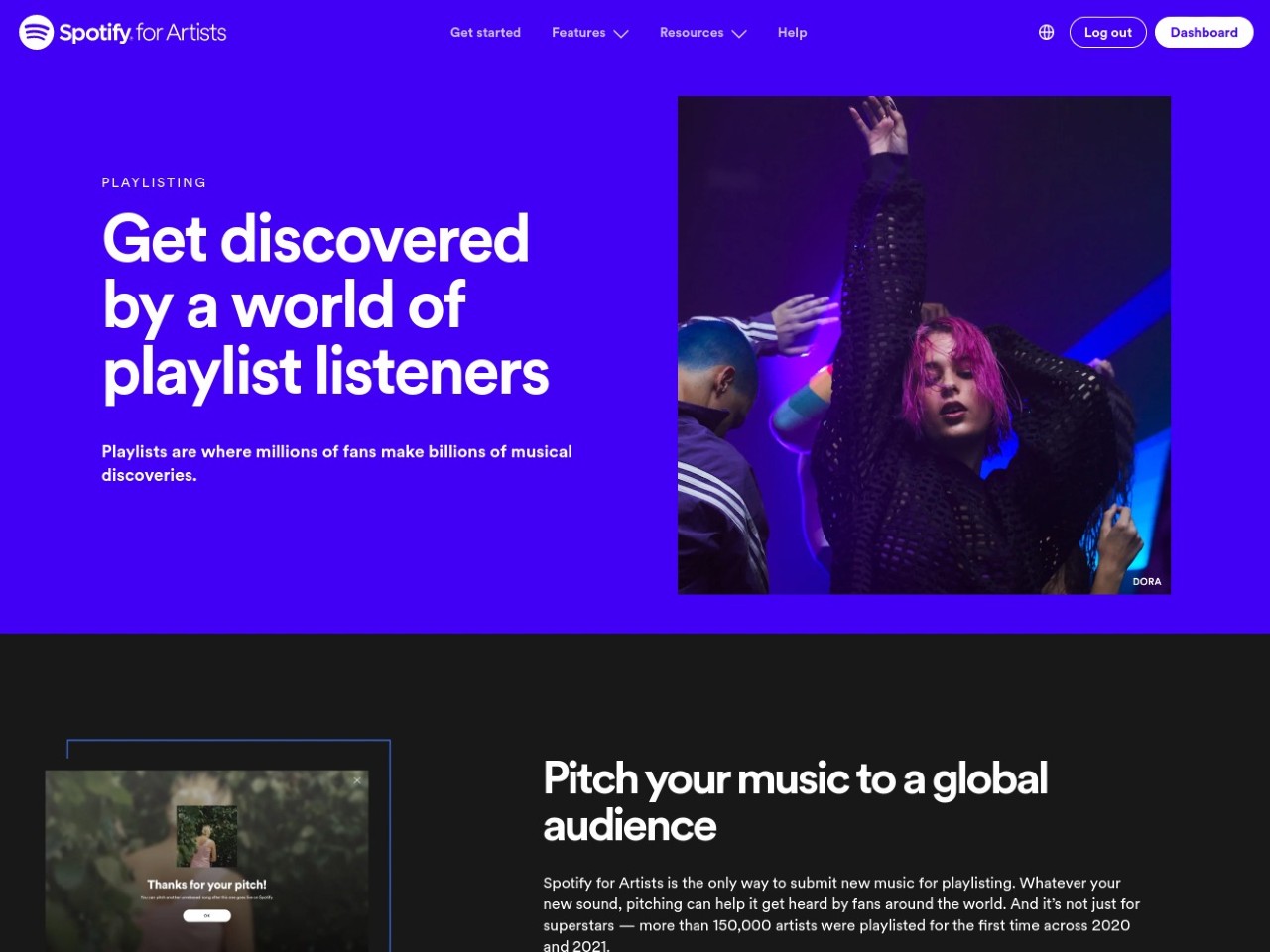Here is a detailed and clean caption for the described image:

---

Screenshot of the Spotify for Artists interface featuring a predominantly blue background. At the top of the interface, navigation options include "Get Started," "Features" with a dropdown arrow, "Resources" with another dropdown arrow, and a "Help" button. On the far-right side, options for "Logout" and "Dashboard" are visible.

Central to the interface is the section titled "Playlisting," with a prominent message saying, "Get discovered by a world of playlist listeners. Playlists are where millions of fans make billions of musical discoveries."

The visual includes an image of an individual dancing joyfully, characterized by pink hair, black clothing, and raised arms, set against a vibrant atmosphere.

At the bottom, against a black background, the text reads: "Pitch your music to a global audience. Spotify for Artists is the only way to submit new music for playlisting. Whenever you pitch new sounds, it can help get heard by fans around the world, not just for superstars. More than 150,000 artists were playlisted for the first time across 2020 and 2021."

Additionally, a side note on the interface says, "Thanks for your pitch."

---